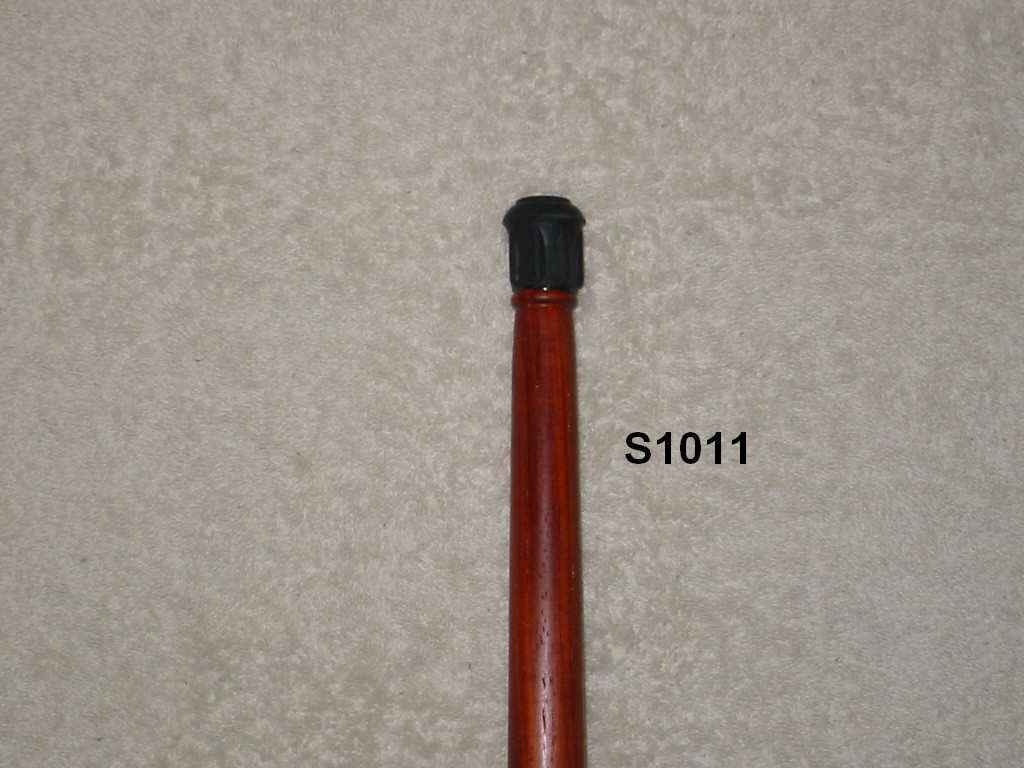This image depicts a close-up of a red-toned, cherry wood grain stick, possibly the bottom of a cane or a similar object, lying against a grayish cement-textured background. The stick, occupying about three-quarters of the photo vertically, features a black, non-skid rubber cap with indentations at the tip. The stick subtly narrows as it approaches the cap, which is securely positioned by an elongated circle near the end. To the right of the stick, there is black lettering that reads "S-1011."